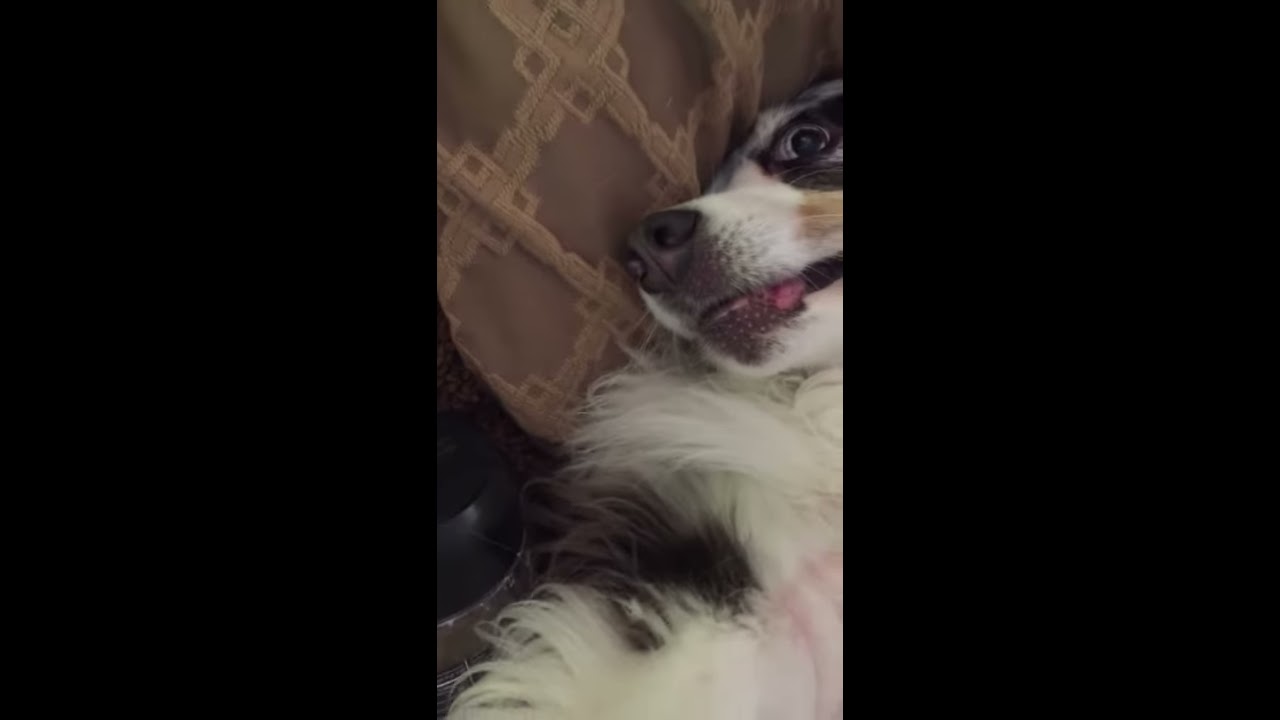In this indoor scene, a dog, possibly a shepherd or collie, is laying on its back with its belly exposed, as if anticipating belly rubs. The dog is centered slightly to the right of the image, with its head turned towards a brown and tan geometrically patterned pillow. The dog appears relaxed, with its mouth slightly open, revealing its top teeth and tongue sticking out towards the left side of its mouth. Its fur is predominantly white with patches of black—most notably around its eyes and the center of its body—with a light brown streak beneath the eyes. Its blackish-brown nose further complements its facial features. The dog is resting on a fabric surface, likely a bed sheet or blanket. In the bottom left corner, the edge of a black shoe or a similar object is visible, though partially cut off, and otherwise, the image is free of other distractions. The color palette includes black, silver, white, pink, gray, red, tan, and light brown, contributing to a warm and cozy atmosphere.